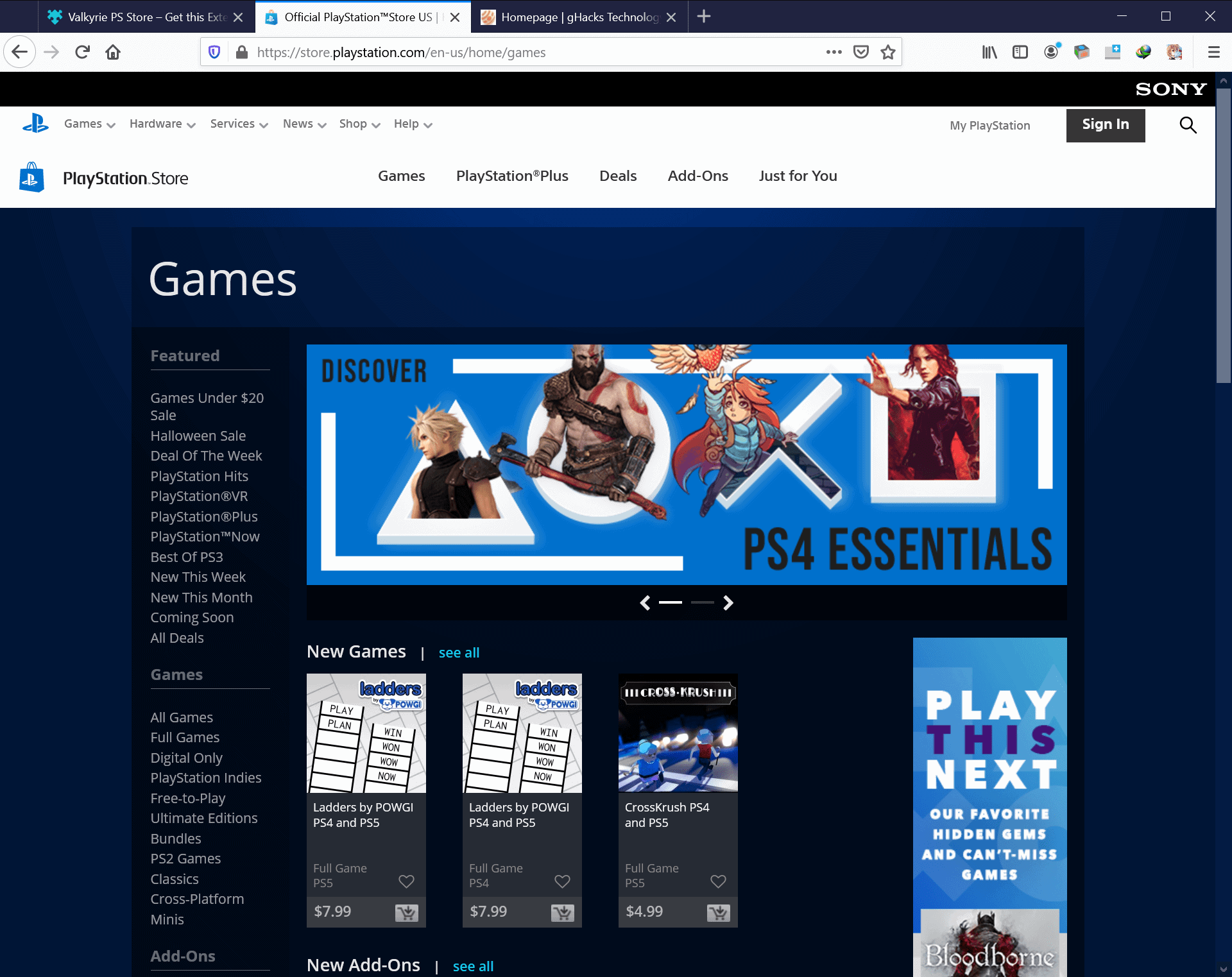A screenshot captured from a computer desktop displays three open tabs at the top of the browser window. The text is small but discernible; the tabs read, from left to right, "Valkyrie PS Store," "Official PlayStation Store," and "Homepage QLLAX Technologies." The active tab is the "Official PlayStation Store," which is the PlayStation website, playstation.com.

In the upper left-hand corner of the page, the PlayStation logo is prominently featured. To the right of the logo, there are six drop-down menus labeled "Games," "Hardware," "Services," "News," "Shop," and "Help." On the upper right-hand corner, the Sony logo is displayed, and right below it, there is a magnifying glass icon. To the magnifying glass's left is a sign-in button, and further left, the "My PlayStation" link is visible.

Directly below the primary PlayStation logo on the left is another PlayStation logo on a shopping bag icon, followed by the text "PlayStation Store." This section offers navigational options including "Games," "PlayStation Plus," "Deals," "Add-ons," and "Just for You." In the screenshot, the user has selected the "Games" option, revealing a list of games currently available on the PlayStation Store.